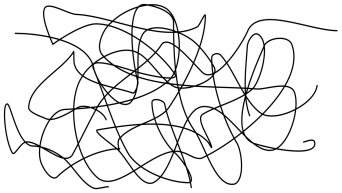The image portrays an abstract piece of art set against a stark white background, dominated by an intricate assembly of black squiggly lines. A singular black line initiates from the top left corner, meandering in a seemingly chaotic fashion across the canvas: it curves down, then swoops upwards, loops around itself within the center, and ultimately vanishes off the screen at the bottom. A similar intricate squiggle begins at the top right corner, curving towards the center and looping around the left side. These lines intertwine to form a visually engaging jumble or messy cluster of random half-loops and swirls. The overall composition resembles a sparse, loosely structured tangle, almost like a disheveled, airy ball of ink marks. Despite the apparent randomness, the lines maintain a sense of fluidity and motion, creating a dynamic abstract artwork approximately an inch to an inch and a half in both dimensions.